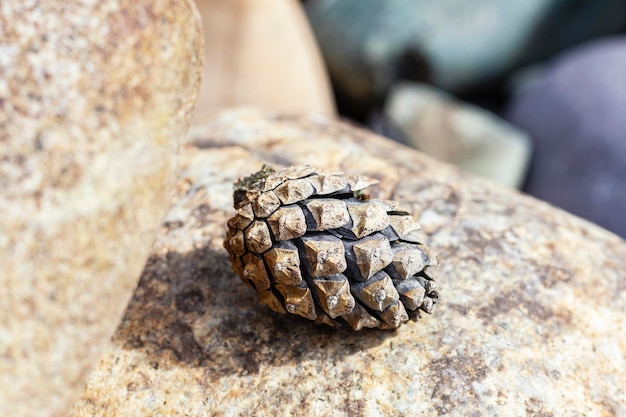In this vivid outdoor photograph, the focal point is a close-up shot of a light brown pine cone, revealing its intricate spikes and curves. The pine cone, with its goldish tan and black hues filling the spaces between scales, rests on a granite-like stone surface. The stone, a blend of light brown and goldish tones with interspersed dark brown shades, extends to the left side of the image, partly obscuring the view. The pine cone's sharp texture contrasts crisply with the smooth, sunlit granite underneath, casting a distinct shadow to its left. The background remains blurred, awash with soft, diffused sunlight, and features an array of colorful stones—one bluish-gray, another purple, and some with cream and yellowish shades—adding to the natural richness of the scene.